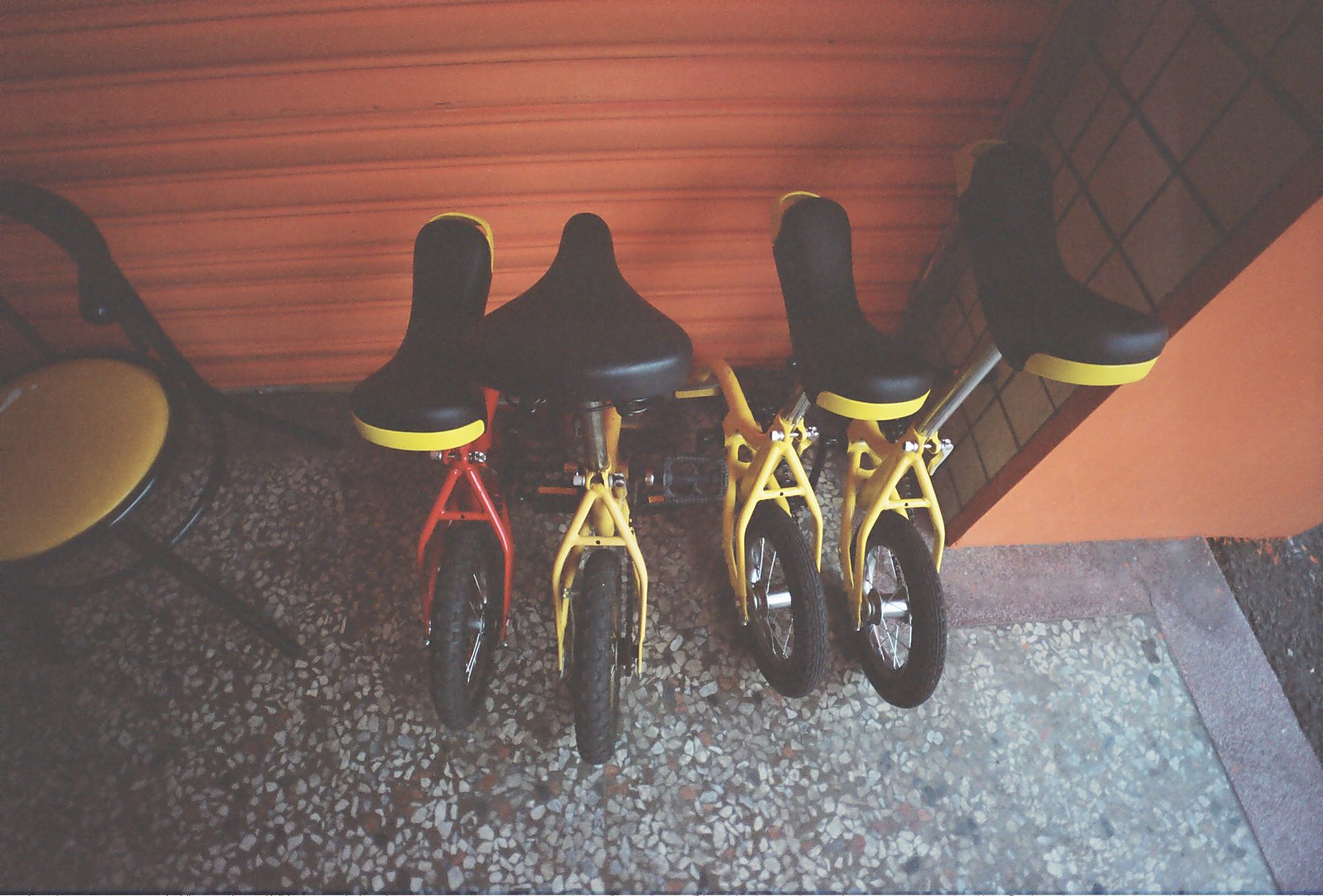This high-quality, landscape-oriented photograph showcases four unicycles parked against a textured, reddish-orange wall, possibly part of a garage opener. Three of the unicycles are primarily yellow, featuring black seats with yellow trim, while the fourth unicycle is distinctively red, also sporting a black seat with yellow edging. The unicycles appear small, likely suitable for children or small individuals, and vary slightly in size. To the far left is a black chair with a yellow seat. The ground beneath the unicycles is speckled, possibly stamped concrete, with some visible asphalt on the right, suggesting a partially outdoor setting.